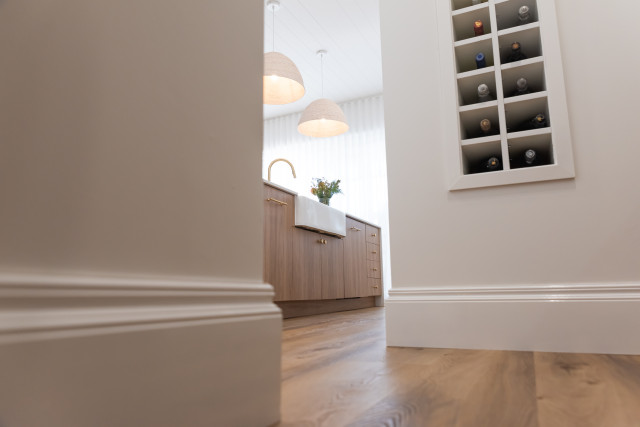This photograph, taken from a low perspective near the floor, captures a domestic kitchen scene. On the left side of the image is a corner wall with a tall, intricate skirting board that transitions into the kitchen area. Dominating the right side of the image is another wall, featuring two columns of small cubby shelves, each holding a bottle of wine. This setup suggests the photo might have been taken from a hallway leading into the kitchen. 

Inside the kitchen, we see a large white sink set into the work units, with a simple, traditional-style gold-colored tap positioned in the backdrop. Dark brown cabinets lie beneath the sink, contrasting with the neutral color palette of the room. A vase of fresh flowers sits next to the sink on the worktop, adding a touch of elegance. Hanging above are two large pendant lights with expansive lampshades, casting a soft glow over the area. The overall decor features neutral tones, including creams and light brown wooden floors, contributing to a premium, sophisticated aesthetic.